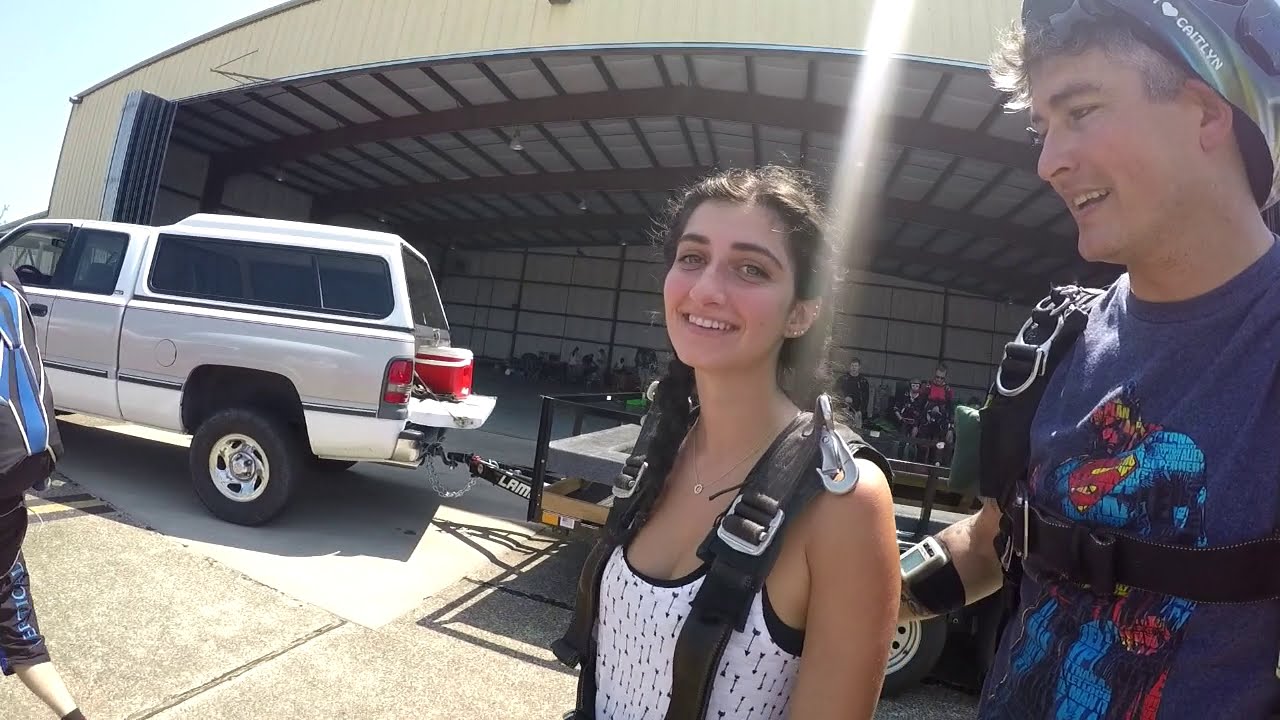This vibrant photograph captures a young couple standing outside a large, bustling hangar, possibly an airplane hangar or a storage facility, filled with lively activity. The woman, with braided dark hair, is beaming at the camera, despite looking slightly tired with mild bags under her eyes. She wears a white tank top and a safety harness equipped with hooks, hinting at an imminent skydiving adventure. Next to her, a man places a supportive hand on her back. He sports a blue t-shirt emblazoned with a Superman logo, a helmet bearing the words "I love Caitlin," and a safety harness. His gaze is fondly directed at the woman. 

A third person, partially visible due to the photo's framing, walks ahead with a backpack. The background is bustling with people also donning harnesses, reinforcing the adventure theme. A large garage or hangar behind them hums with activity; people inside appear to be gathered around a truck pulling a trailer. The brightly lit scene suggests a vibrant, possibly celebratory atmosphere, as if the couple is on the cusp of an exhilarating skydiving experience.